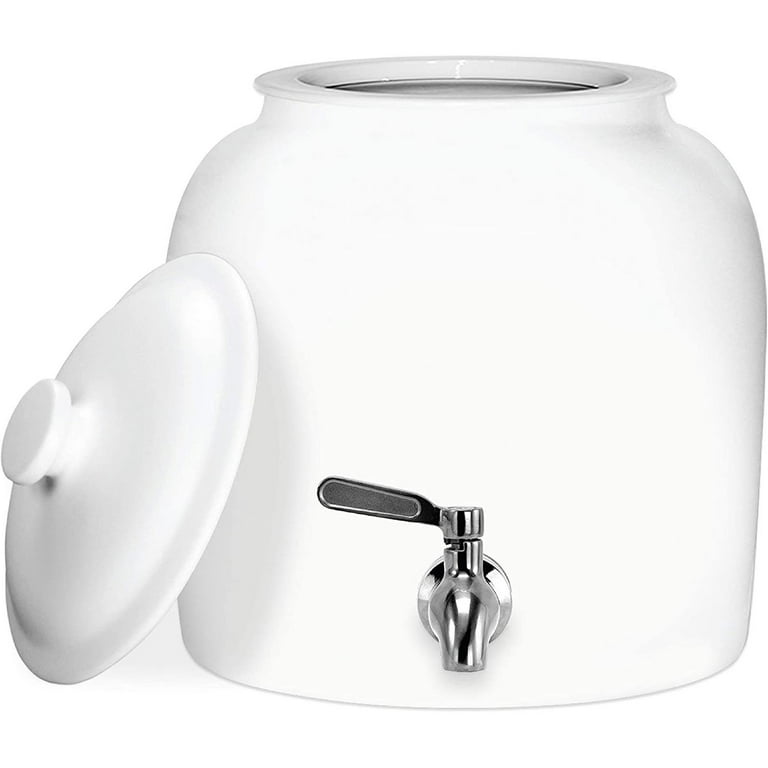The image captures a simple, unadorned white ceramic pot set against a plain white background, with no borders or additional elements. The pot has its removable lid off and leaning against its left side, casting a shadow. This minimalistic container features a silver metal spigot at the center bottom, equipped with a turn handle for dispensing liquids stored within the pot.